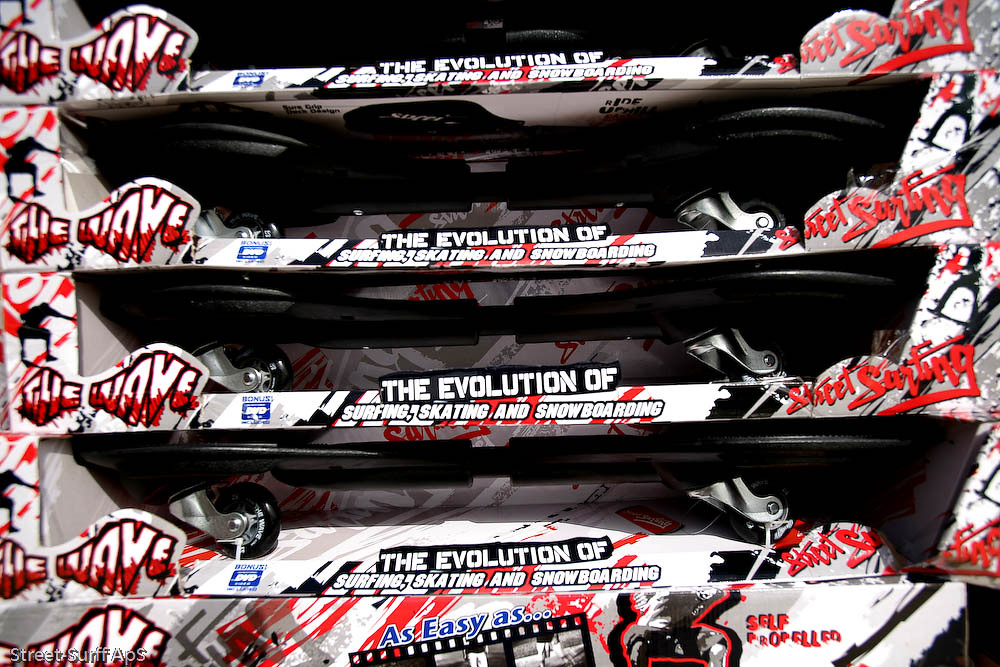This image depicts a sporting goods store display that prominently features four identical rectangular boxes stacked vertically, each containing a skateboard-like device. The boxes are primarily decorated with black and white text and images, including a notable phrase in white letters that reads, "THE EVOLUTION OF SURFING, SKATING, AND SNOWBOARDING," set against a black background. On the left side of the display, there is a sign with the word "MOVE" printed in white against a black backdrop. Each box includes a skateboard-like device with two wheels connected by a rod, which allows it to twist, resembling a wave. There is also red text on some parts of the packaging, mentioning "street surfing." Additionally, there are gray hats visible within the display, suggesting a variety of related merchandise. A blue "BONUS DVT" symbol appears at one side of the boxes, adding to the colorful array of branding elements. The repetitive design and clear emphasis on the evolution of action sports encapsulate the dynamic nature of the products featured in this sporting store.